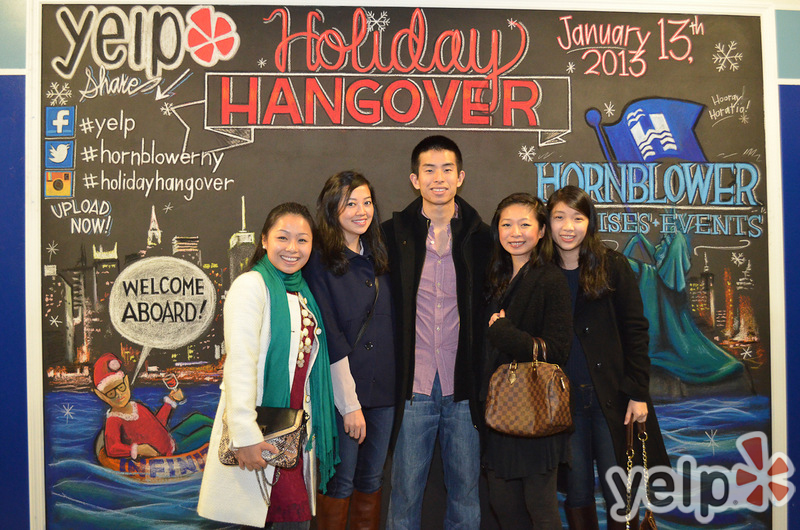In this vibrant photo, five smiling young people, all appearing to be of Asian descent, are closely grouped together, standing in front of a lively and artistic backdrop. The setting is festive, marked by a large hand-drawn chalkboard illustration announcing a "Yelp Holiday Hangover" event, which took place on January 13th, 2013. The backdrop features a whimsical scene with a skyline beside a body of water, a floating Santa Claus holding a wine glass with a red beverage, and various festive elements. The Santa figure on a life preserver says "Welcome Aboard" in a speech bubble. Surrounding the scene are well-known social media icons for Facebook, Twitter, and Instagram, alongside hashtags and messages like "Upload Now." At the bottom right, the Yelp logo is prominently displayed. Text on the backdrop also includes "Hornblower Events," hinting at the event's organizer. The group composition includes two women on the left, a man in the center, and two women on the right, all looking cheerful and happy, capturing a moment of joy and camaraderie.